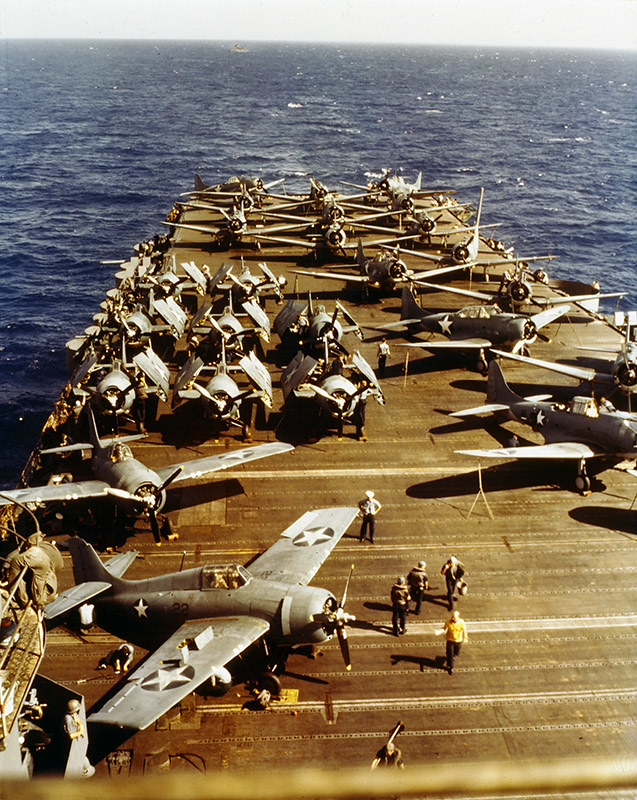The image is a vintage wartime photograph showcasing an aircraft carrier deck populated with numerous warplanes. The photograph, tinted with a yellowish hue from age, captures about 20 to 25 silver, propeller-driven airplanes, each bearing a blue circle with a white star insignia on their wings. The front plane is prominently featured, facing right, surrounded by men in various activities. Behind it, planes are orderly arranged in rows—some with wings folded upwards and others extended. The aircraft carrier, rectangular in shape, is in a choppy blue ocean, beneath a light gray sky. The scene is bustling with personnel on deck, and horizontal lines are visible across the platform. The distant water appears rocky, emphasizing the maritime setting.